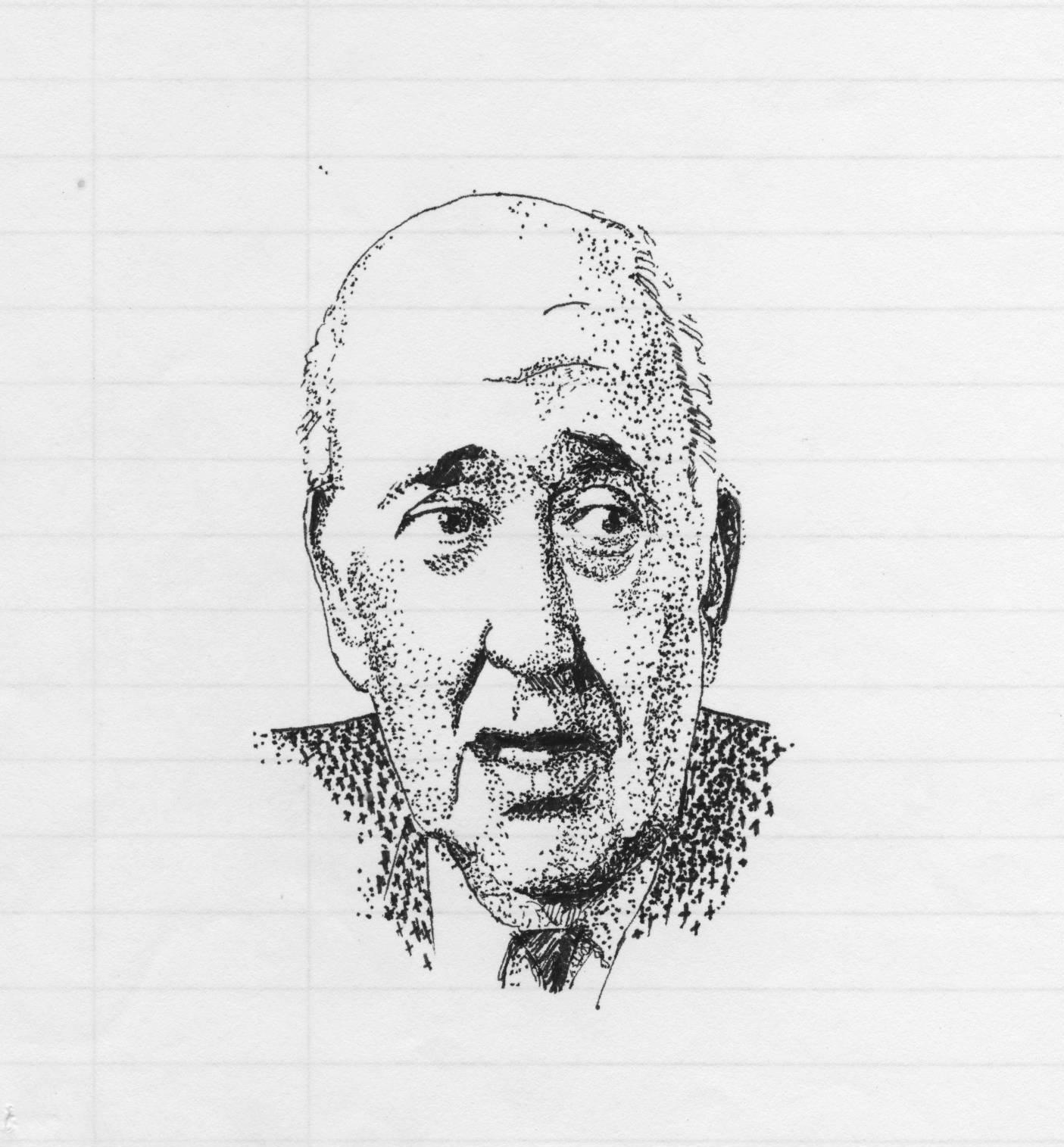This black and white image is drawn using a technique called stippling, made mostly of dots and very short lines. It appears on lined loose-leaf paper, identifiable by horizontal lines and two vertical lines on the left margin, indicative of a notebook page. The drawing depicts an older, bald man with some hair on the sides of his head. He is depicted in a frontal view with his eyes glancing towards the right side of the image. His facial features are detailed: ears, nose, and slightly open mouth suggest he might be in the middle of speaking. He is dressed in formal attire, consisting of a suit jacket, a button-down shirt, and a tie. The image focuses on his head, neck, and the upper part of his shoulders, framed in a square format against the lined paper background.